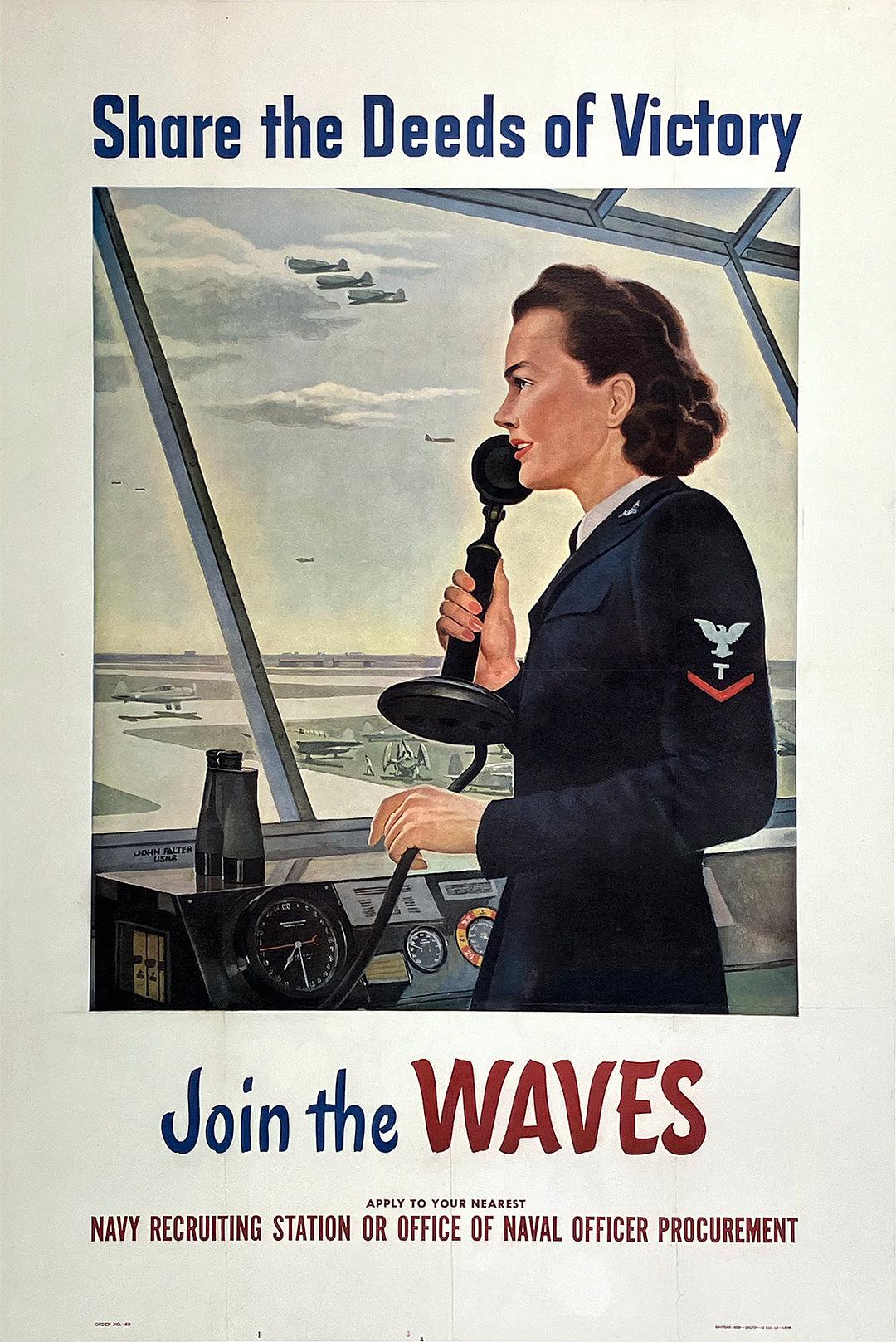This World War II-era Navy recruitment poster features a detailed illustration set against an off-white background. At the top, in bold blue letters, the poster reads, "Share the Deeds of Victory." Below, a woman in a blue Navy uniform, adorned with a white eagle, a "T," and a red insignia on her left arm, holds an old-style black microphone up to her mouth. She stands within what appears to be a control tower, surrounded by a machine instrument with circular gauges and dials, and a pair of binoculars resting nearby. The background includes a runway with a stationary airplane, and the sky above features three planes flying in formation among white clouds. Below the illustration, in mixed blue and bold red text, the poster urges, "Join the WAVES," emphasizing the acronym in red. At the bottom, the call to action reads, "Apply to your nearest Navy recruiting station or Office of Naval Officer Procurement," in red text.